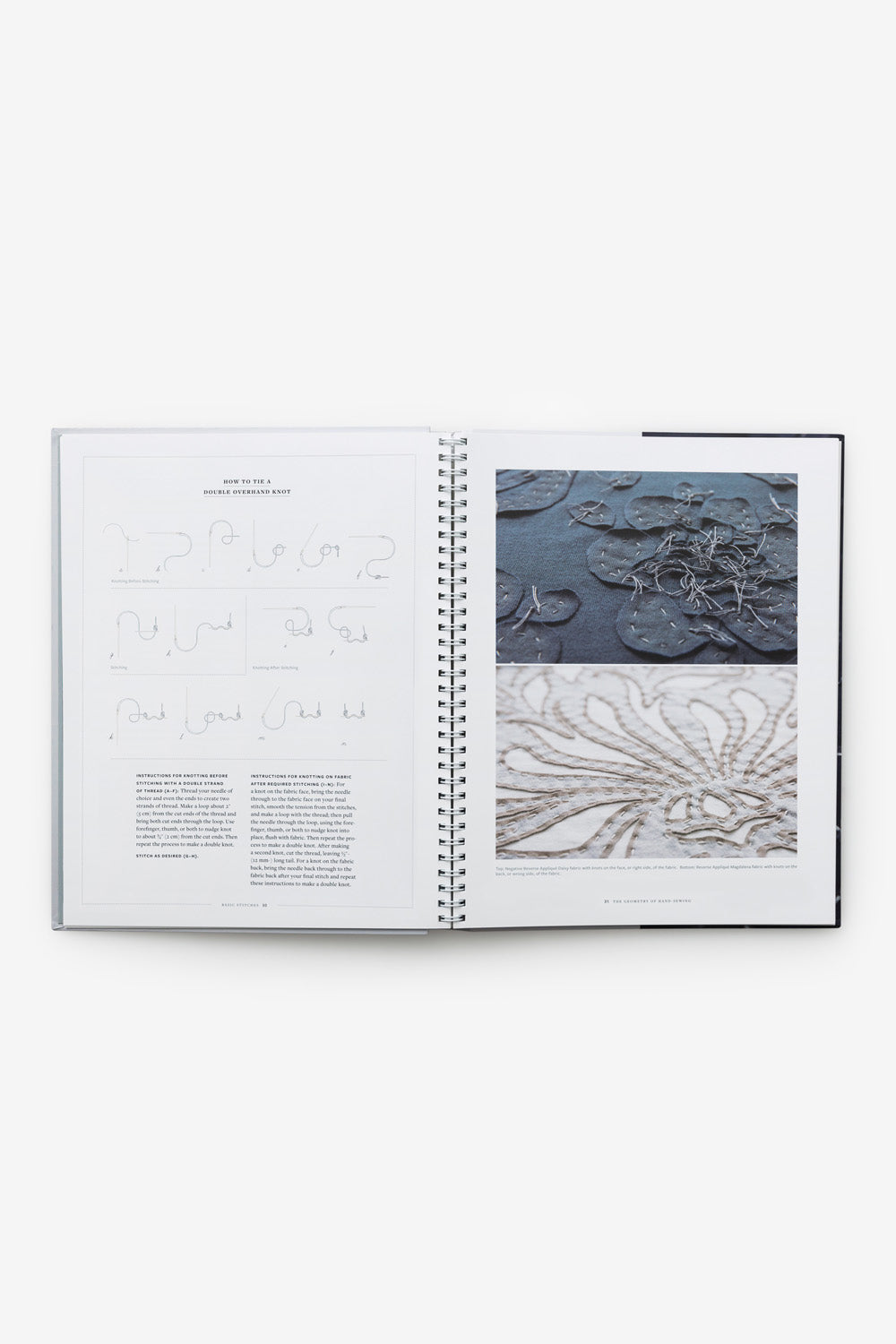The image depicts an open spiral-bound notebook lying flat on a surface. The pages are white with a mix of text, illustrations, and photographs. On the left page, there is a block of handwritten text accompanied by indiscernible pencil drawings or squiggly lines. These illustrations don't represent anything specific. The right page showcases two black-and-white photographs. The top photograph presents indistinct grayish-brown objects that appear to be in mud, possibly shells. The bottom photograph is a close-up of the objects from the top photo, highlighting their intricate and intriguing designs. The notebook's hardcovers are gray on the left and dark gray or black on the right, giving it a professional and sturdy appearance.